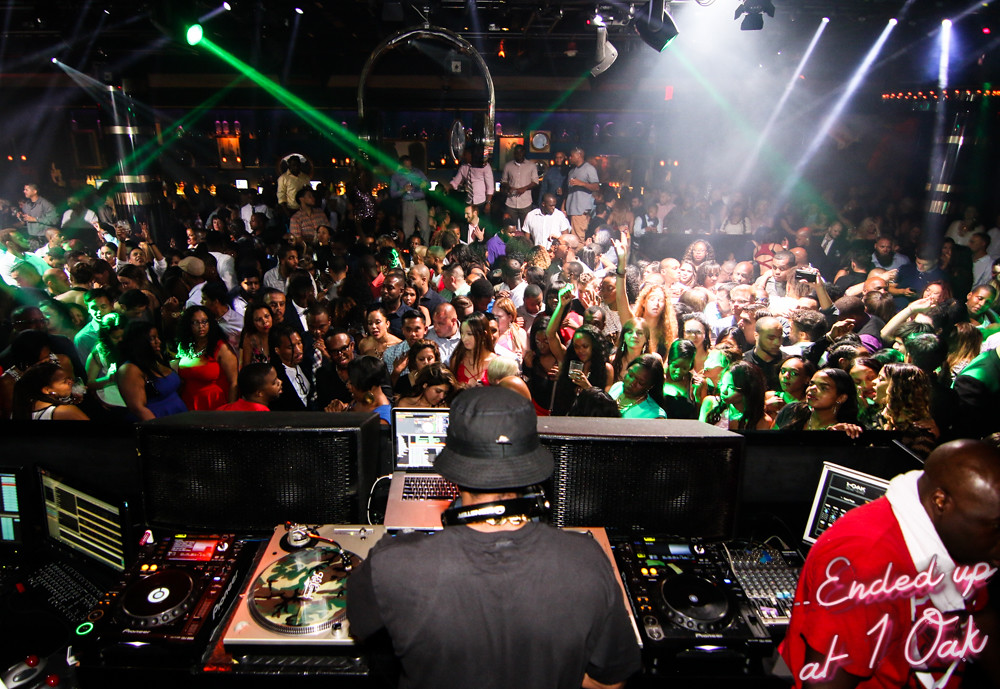In this vibrant nightclub scene, a DJ dressed in a black t-shirt and black bucket hat commands the decks at the bottom center of the image. Just in front of him lies a pair of turntables and a laptop, signifying his craft. Adjacent to the DJ stands a man in a red t-shirt with a white towel draped over his shoulder. A diverse and energetic crowd fills the top portion of the frame, predominantly composed of young men and women, many of whom are dancing, taking pictures, or raising their hands in excitement. The background is adorned with dark hues and punctuated by vibrant lights—green, white, and other colors—emanating from the ceiling and creating a laser-like effect. Large speakers flank the walls, enhancing the pulsating atmosphere. The text "Ended Up at One Oak" is visible in the bottom right corner, anchoring the scene to the renowned nightclub.